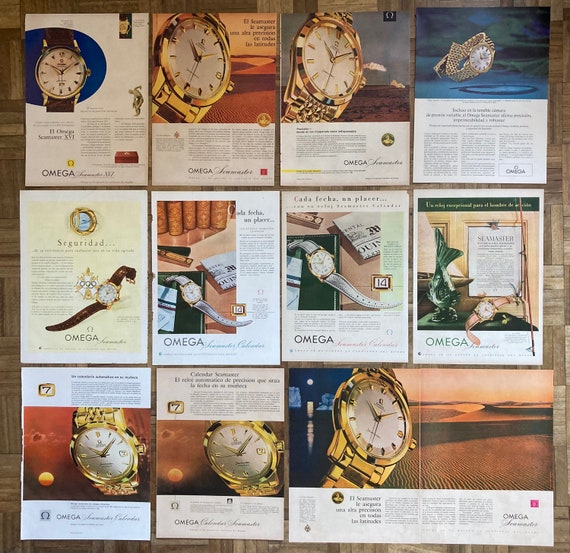The image depicts a collection of 11 advertisements for Omega watches, resembling a magazine layout or possibly vintage promotional material. The advertisements are arranged in a grid-like fashion against what appears to be a brown wooden surface, possibly a floor. Each ad showcases the elegant, high-end timepieces in vivid detail, with some featuring close-ups of the watch faces and others displaying the full watch including the bands, which vary from gold to leather. Despite the small print, the Omega branding is discernible, indicating the luxury nature of these watches. The range includes larger men's watches on the bottom and medium-sized ones in the middle that could be unisex, with a daintier lady's watch positioned at the upper right. The overall presentation of the advertisements is quite detailed, emphasizing the classy and slightly varied designs of each watch, all depicted in color ads with plentiful text. The overall impression is one of timeless sophistication and meticulous craftsmanship.